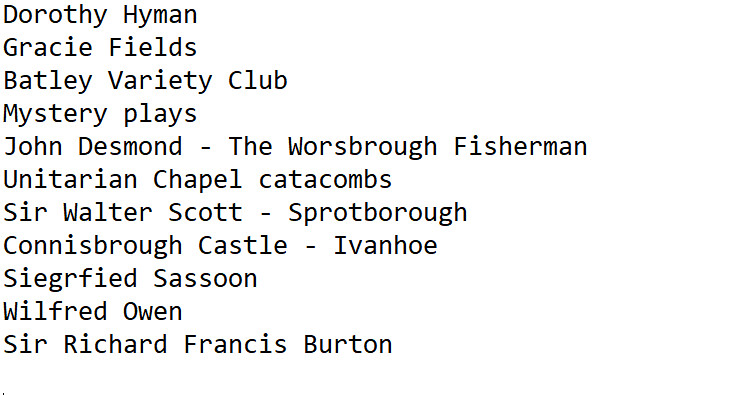The image features a minimalist black-on-white list, formatted like typewriter text, with eleven lines of names and titles, all left-aligned. The list includes notable British figures and places such as athlete Dorothy Hyman, singer Gracie Fields, the Batley Variety Club, the phrase "Mystery Plays," John Desmond referred to as "The Warsboro Fisherman," the "Unitarian Chapel Catacombs," author Sir Walter Scott associated with "Sprottboro," "Conniesboro Castle - Ivanhoe," poet Siegfried Sassoon, poet Wilfred Owen, and explorer Sir Richard Francis Burton. The context or connections between these names and titles are unclear, resembling perhaps an invitation or program listing.